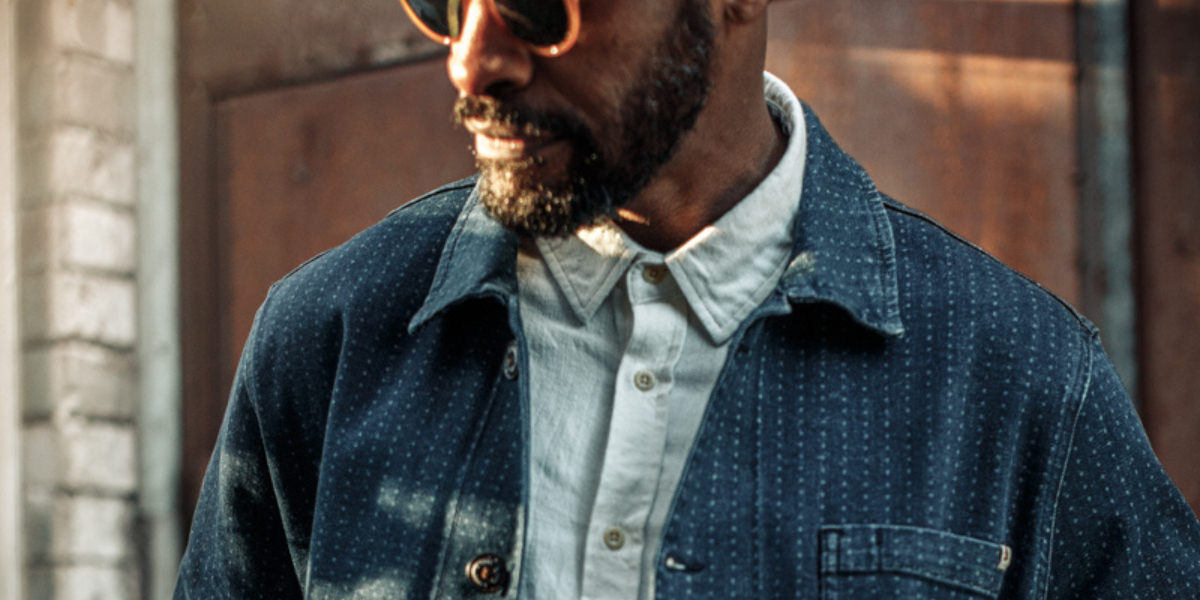This tightly cropped photo captures an African-American man from his eyes down to mid-torso. He has medium dark skin, a full beard with flecks of gray, and a mustache that connects with his beard. The man sports orange-rimmed sunglasses with black-tinted lenses and wears a navy blue jacket adorned with orderly, white polka dots, contrasting with its dark color. Beneath, he has a light blue button-up shirt fastened completely up to its collar, featuring grey buttons. In the background, a residential setting is slightly blurred, showcasing wooden panels, a dark-stained door, and white brick elements. Sunlight from the left illuminates his face, adding a fashionable flair to his composed stance.